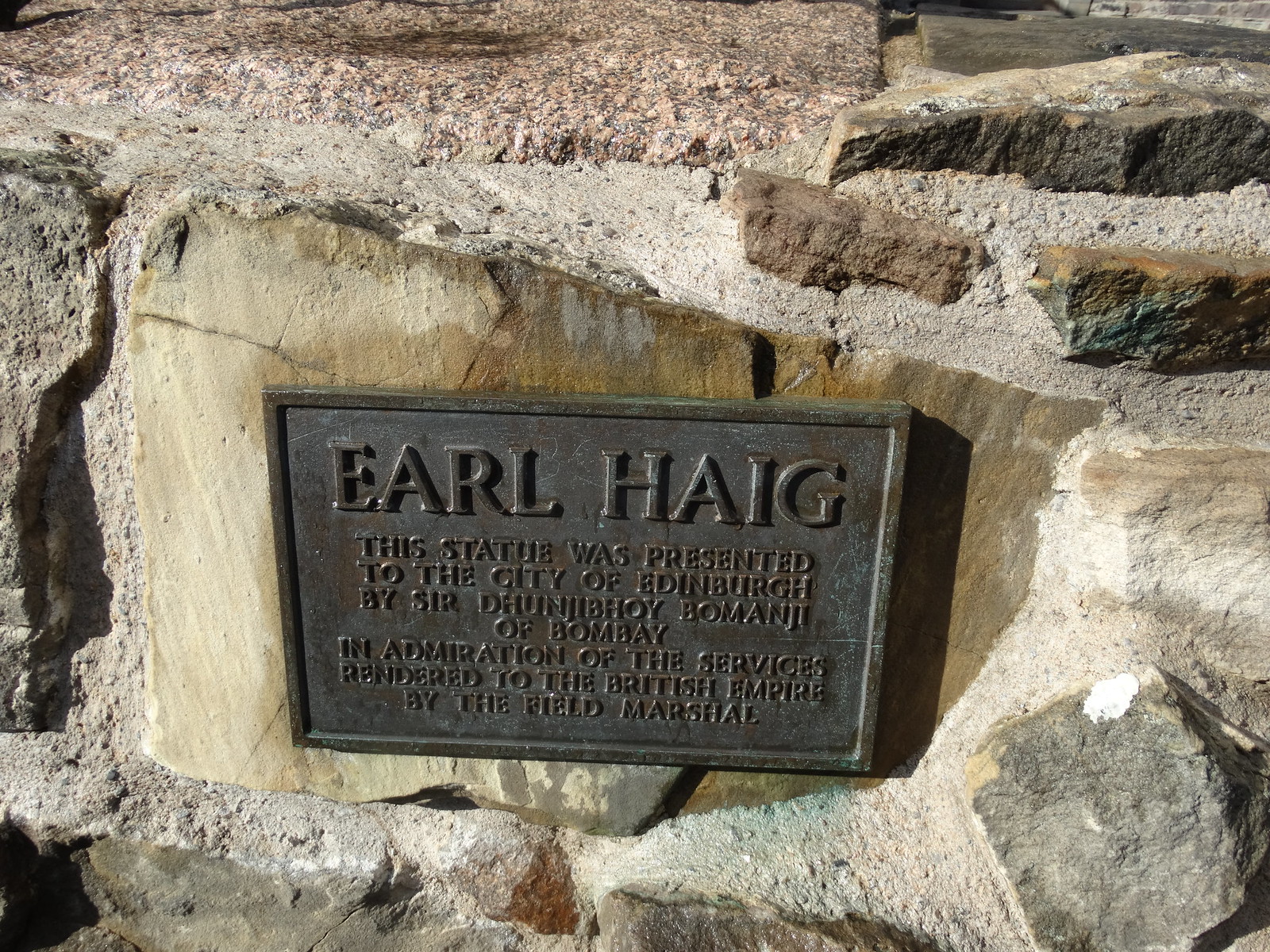The plaque is installed within a varied stone and cement wall composed of multi-colored rocks, predominantly in shades of brown and gray, with some appearing off-white and possibly granite or marble. The dark gray metal plaque is adorned with prominent raised lettering at the top that reads "Earl Haig," H-A-I-G. Beneath this in etched text, it declares: "This statue was presented to the city of Edinburgh by Sir Bibi Bomanji of Bombay in admiration of the service rendered to the British Empire by the Field Marshal." The detailed inscription highlights the plaque's commemorative purpose, honoring Field Marshal Earl Haig, likely dating from the late 19th to early 20th century. The plaque evidently situates at the base of the statue, contributing to its historical significance.